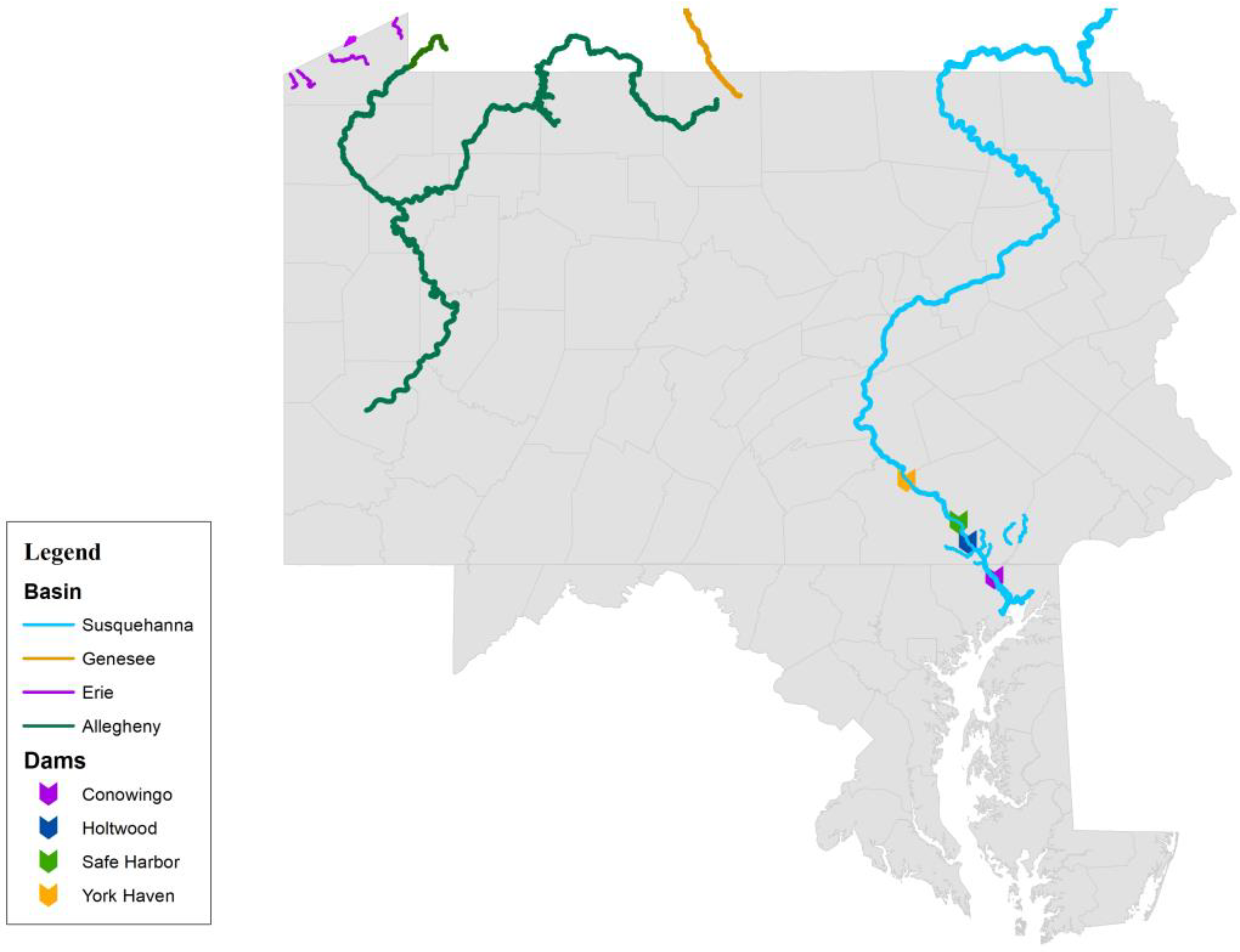This is a detailed gray map featuring the states of Pennsylvania, Maryland, and New Jersey, with no clear boundaries between them. The map highlights various rivers in distinct colors: dark green, purple, yellow, and a prominent turquoise. The turquoise river is marked with chevron symbols indicating dams, specifically the Conowingo, Holtwood, Safe Harbor, and York Haven dams, as per the legend. The legend is divided into two sections: basins and dams. The basins listed include the Susquehanna River, Genesee River, Erie River, and Allegheny River. The entire image is outlined in black and is presented in high quality, making it evident that this map is focused on depicting watershed information.